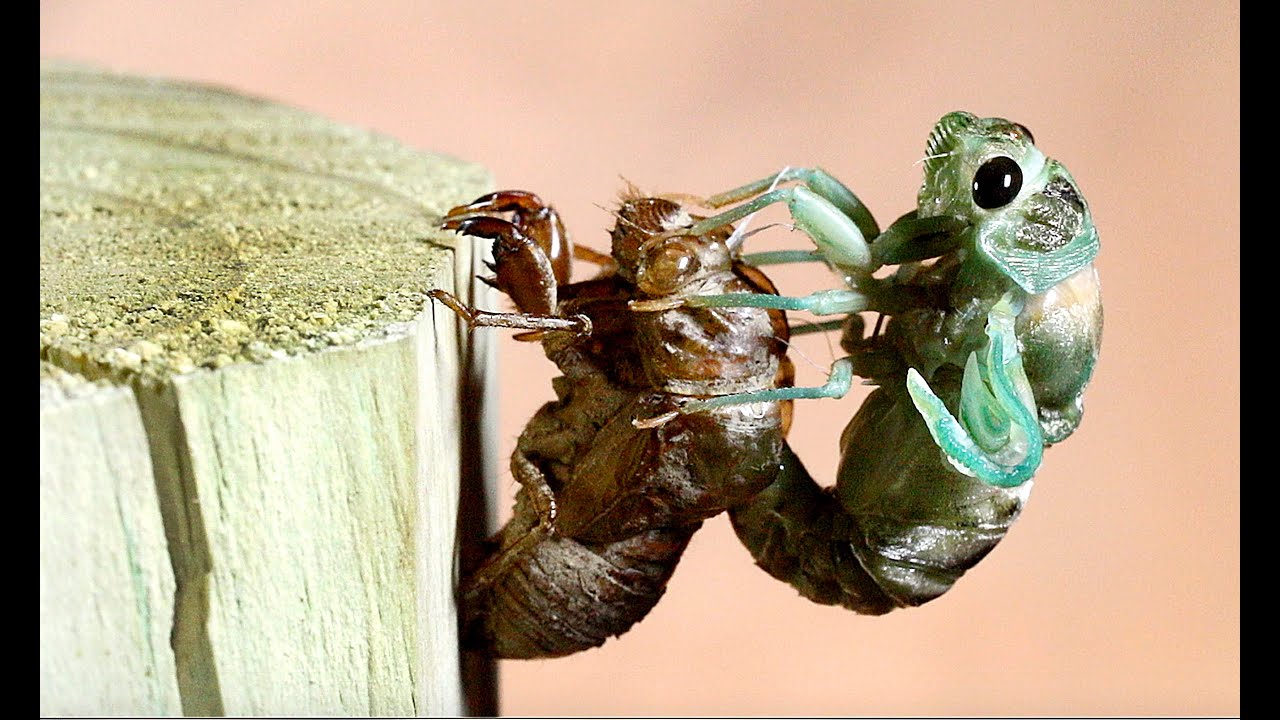The image depicts a detailed scene of a molting insect, likely a cicada, in the process of emerging from its exoskeleton. The insect on top has a striking teal color with dark gray and brownish hues, featuring prominent black eyes. Its legs are wrapped around the exoskeleton of the insect below, which is a brownish color and appears to be firmly attached to a cut-down branch or log. The background features a pink hue, contrasting with the predominantly white log. The emerging insect's wings are still curled up, indicating its freshness and the immediacy of its molting process. This gives a vivid portrayal of the natural transformation from the exoskeletal shell to its new form.